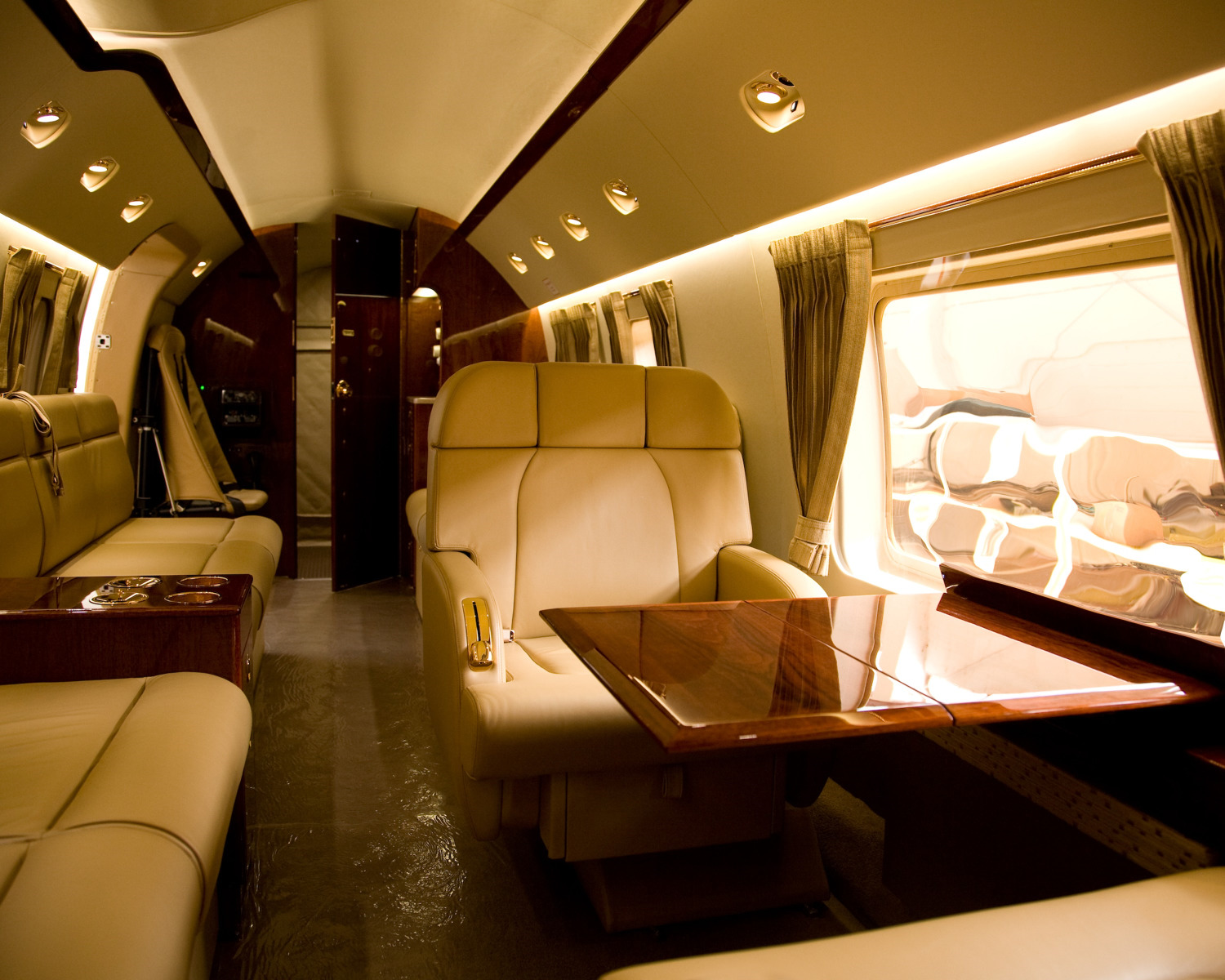The photograph depicts the luxurious interior of what appears to be a first-class section of a train or possibly a tour bus. The left-hand side prominently features a series of tan-colored cushioned bench seats, divided by a sophisticated brown barrier that includes functional cup holders. Adjacent to these seats stands an elegant, overstuffed tan recliner chair, positioned beside a brown table that gleams under the light streaming in from a large window. The window is flanked by rich drapes pulled back to allow an unobstructed view outside. Behind the recliner and table setup lies another similar window, complete with matching drapes. As the scene extends to the rear, we notice another tan-colored booth seat positioned on the left, facing a dark brown entryway that subtly beckons from the background. The ceiling above showcases a harmonious blend of dark browns and dark yellows flanking a lighter brown-colored ceiling tile through the center, completing the opulent and inviting ambiance of the space.